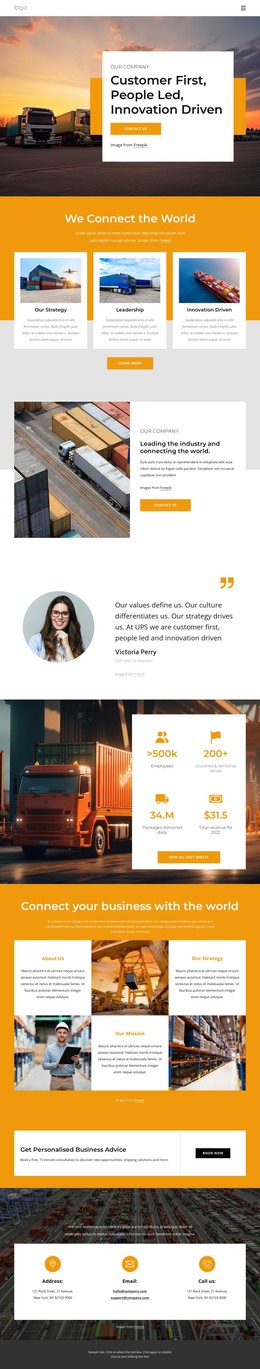A screenshot of a long webpage, potentially captured using Firefox's full-page screenshot feature, appears distorted with overly compressed dimensions, making its content nearly illegible. At the top of the page, there is an image of a sunset behind several semi-trucks accompanied by the text: "Customer First, People Led, Innovation Driven" and a yellow button. Below this, a yellow box reads: "We Connect the World."

Further down, the page showcases three images, seemingly depicting an airplane hangar, a semi-truck, and a cargo ship. A yellow button is positioned underneath these images. An aerial view, presumably captured by a drone or helicopter, displays a yard filled with shipping containers, accompanied by another yellow button.

Centrally located on the page is a circular image of a long-haired individual, potentially a woman, though the facial features and potential glasses cannot be clearly discerned. There are quotation marks with unreadable black text next to this image. Below, another image of a semi-truck is featured with four golden icons, though the text associated with these icons, including terms like "5000K" and "200," cannot be deciphered.

Further down, a yellow background frames three additional images: one possibly showing a person with a clipboard, another potentially the underside of a railway bridge from a low angle, and the last resembling a view inside a Costco store as if seen from a wheelchair. The page concludes with three more orange icons or sections, the purpose of which remains unclear due to the image's distortion.